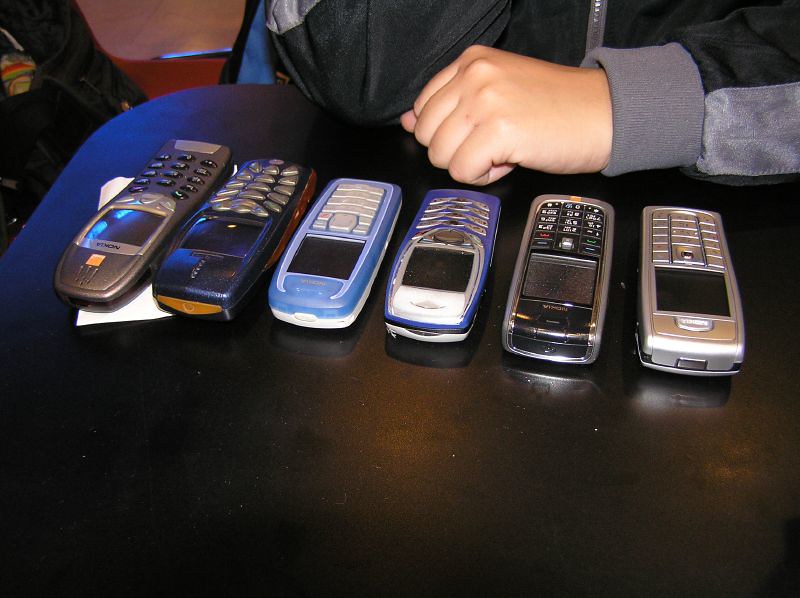In this image, six older Nokia cellphones are neatly arranged on a brown table that has a subtle glare from a light source. The phones, which are all turned off, are positioned with their tops facing the bottom of the photo and their bases towards the top. Each phone displays a unique design:

1. A dark gray phone with black buttons and a slightly larger screen.
2. A black phone with a yellow port at the top and gray buttons.
3. A small phone with a blue front, a white back, and white buttons.
4. A dark blue phone featuring gray buttons and a white section at the earpiece.
5. A silver phone with black buttons that either illuminate or have white text.
6. A completely silver phone with matching silver buttons.

Across the table, a person is visible, clad in a black jacket with gray stripes along the sleeve and a gray-cuffed pocket. This person has their fist resting on the table. There's also a hint of an indistinguishable tan-and-brown item in the left corner, possibly a backpack. The entire scene captures a nostalgic array of classic cell phones with a hint of human presence in the background.